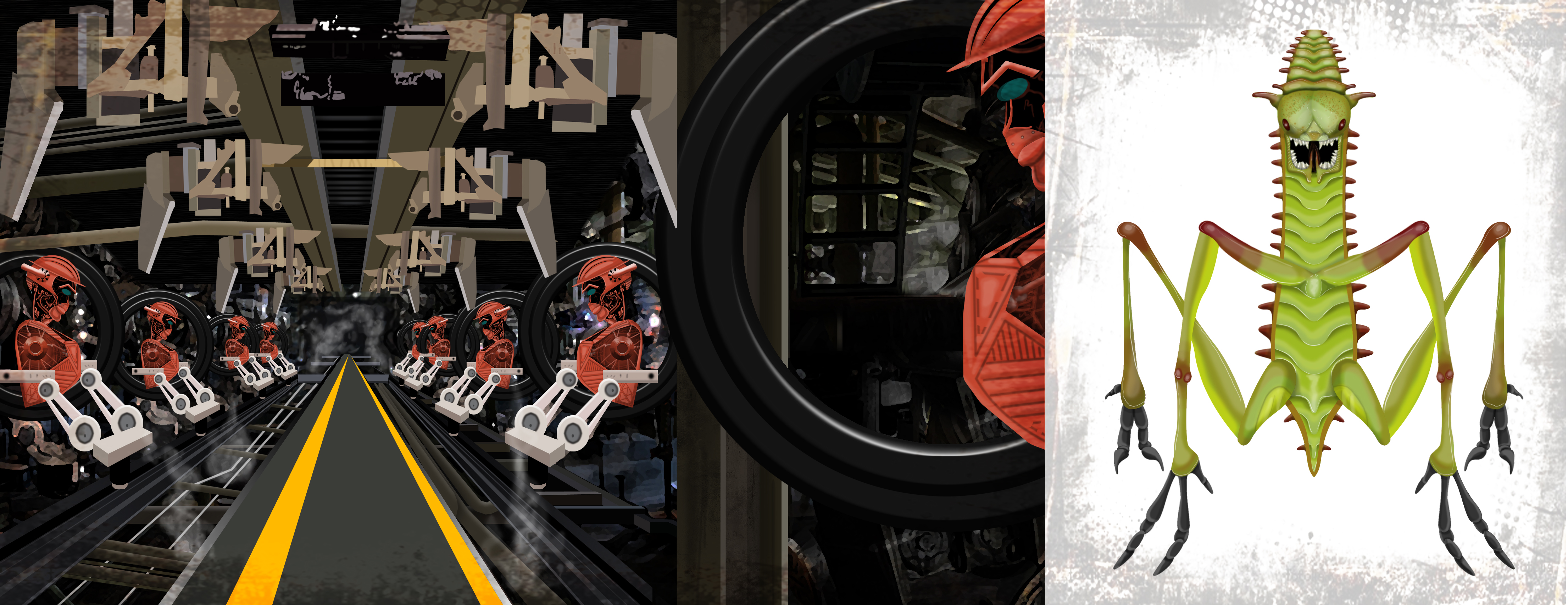The image comprises two separate artworks displayed side by side. On the left, there is a computer-generated scene resembling a factory or a military transport setup. Central to this scene is a black conveyor belt with two orange stripes, flanked on either side by four red robots possessing white arms, totaling eight robots. These robots, which could be perceived as game characters, are seated in pairs across the conveyor belt, perhaps preparing for an imminent mission. An additional red robot is positioned on the right side of this scene, seemingly peering around a corner towards the central conveyor area.

On the right, the scene contrasts sharply with the depiction of a monstrous creature. This green, grasshopper-like monster exhibits reptilian features and is set against a white background framed by gray. The creature's menacing open mouth reveals sharp, formidable teeth, and its appearance is enhanced by dark brown accents and a scaly texture. It's a fantastical, fearsome insect-like entity with four limbs, each ending in claws characterized by a set of three toes, two of which are notably elongated.

Overall, the juxtaposition of these two scenes suggests a narrative where the team of red robotic figures on the left might be embarking on a mission to confront or eliminate the vicious green monster on the right.